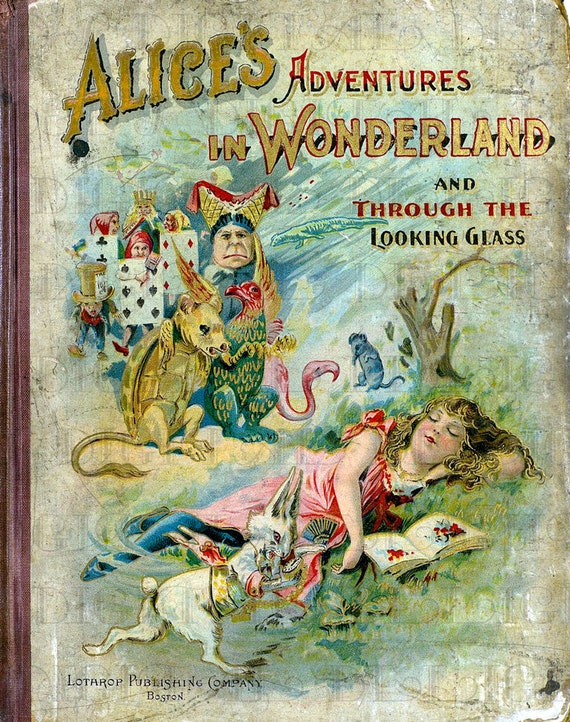The image captures an aged, well-worn book cover of "Alice's Adventures in Wonderland and Through the Looking-Glass," published in Boston by Lotharop Publishing Company. The title at the top is rendered in a mix of gold, red, and black lettering, prominently displaying the book's name. The cover is a greenish tint and shows signs of wear, with torn and discolored edges, especially evident in the upper corners.

Central to the cover is a colorful illustration featuring several iconic characters. In the lower right corner, Alice, depicted with golden hair, is laying on a grassy hill wearing a pink or red dress, blue tights, and appears to be napping. In the lower left corner, the famous white rabbit is seen running towards the right. Above Alice and to the left, there are playing cards with faces, representing the anthropomorphic card characters from the story. There's also a man with a decorative headpiece, a monster-like creature with the body of a turtle, a lion's tail, and a head resembling a rat or mouse, and a bird, all situated in the upper left-hand corner. The spine of the book, visible on the left side, is brown and contributes to the overall vintage appearance of the cover.